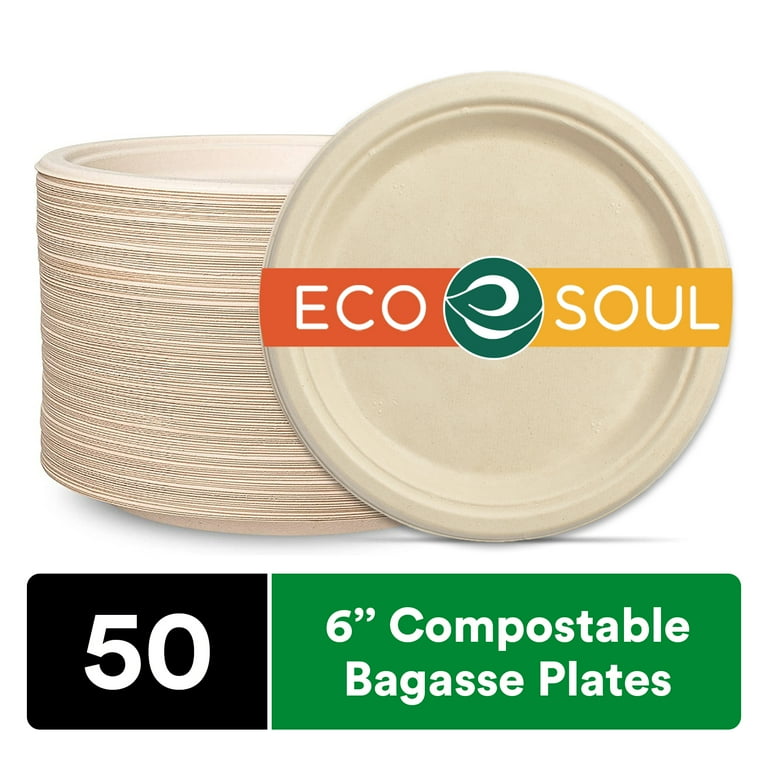The image is an advertisement for recyclable, compostable 6-inch bagasse plates. On the left side, there is a stack of approximately 50 green plates. Adjacent to the stack is a single plate, positioned vertically on its edge, showcasing the top side of the plate. Across the front of this plate, a vibrant graphic prominently displays the text "Eco Soul" in white, set against an orange and yellow background with a green circle in the center, containing a white swirl. At the bottom of this graphic, a black background features the text "50" in white, indicating the quantity, while a green background below that specifies "6 inch compostable bagasse plates." The plates appear to be packaged together in plastic, with the branding clearly visible.